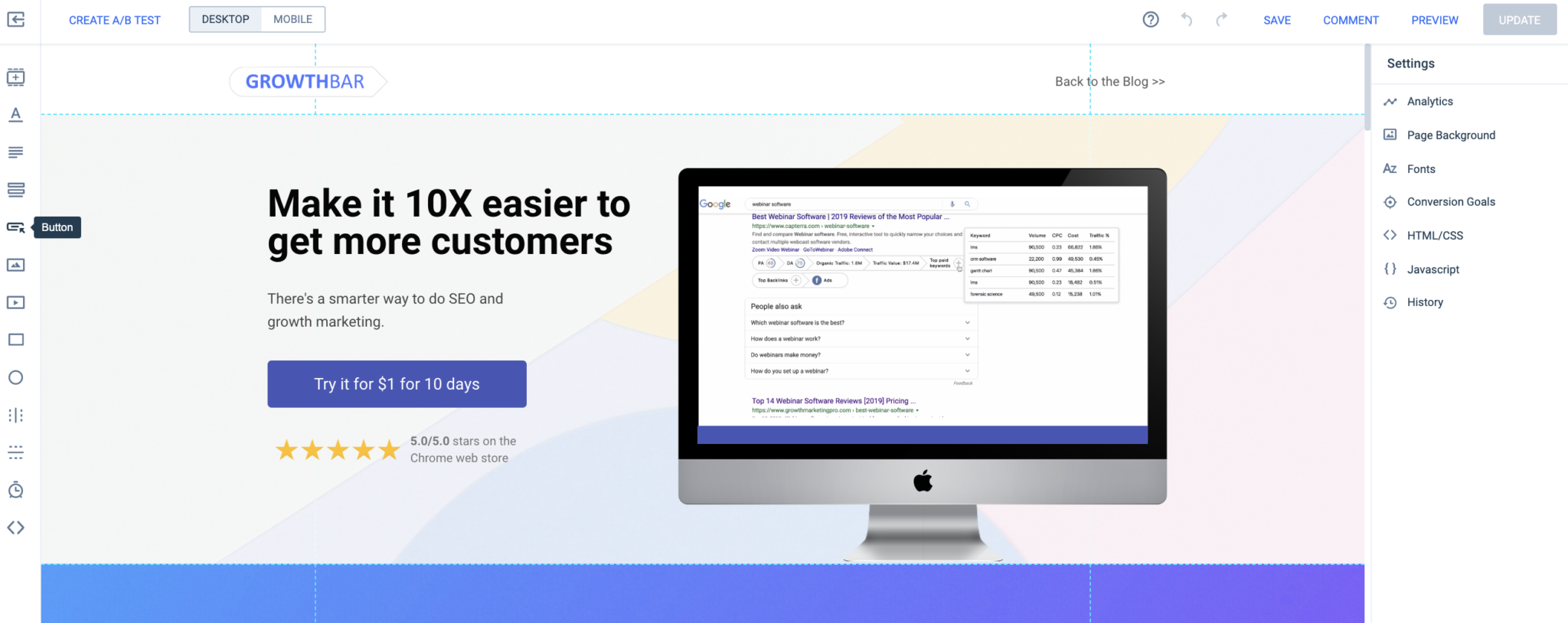The image depicts a webpage divided into three main sections, each flanked by two side panels. The left side displays various icons, the meanings of which are unclear. The right side panel lists several options, including settings, analytics, page background, fonts, conversion goals, HTML, JavaScript, and history.

The central section features a prominent call to action for creating an A/B test, with options to choose between desktop or mobile; in this case, desktop was selected. Below this, there is a promotional message about a tool called "Growth Bar," which claims to make it ten times easier to acquire more customers, offering a trial for $1 for 10 days.

The page touts itself as a smarter solution for SEO (Search Engine Optimization) and growth marketing. The background is gray, and there is an image of an Apple iMac or monitor displaying a Google search result page, reinforcing the focus on improving search engine rankings and online visibility. The tool appears to offer features aimed at enhancing SEO performance to achieve better ratings on search engines.